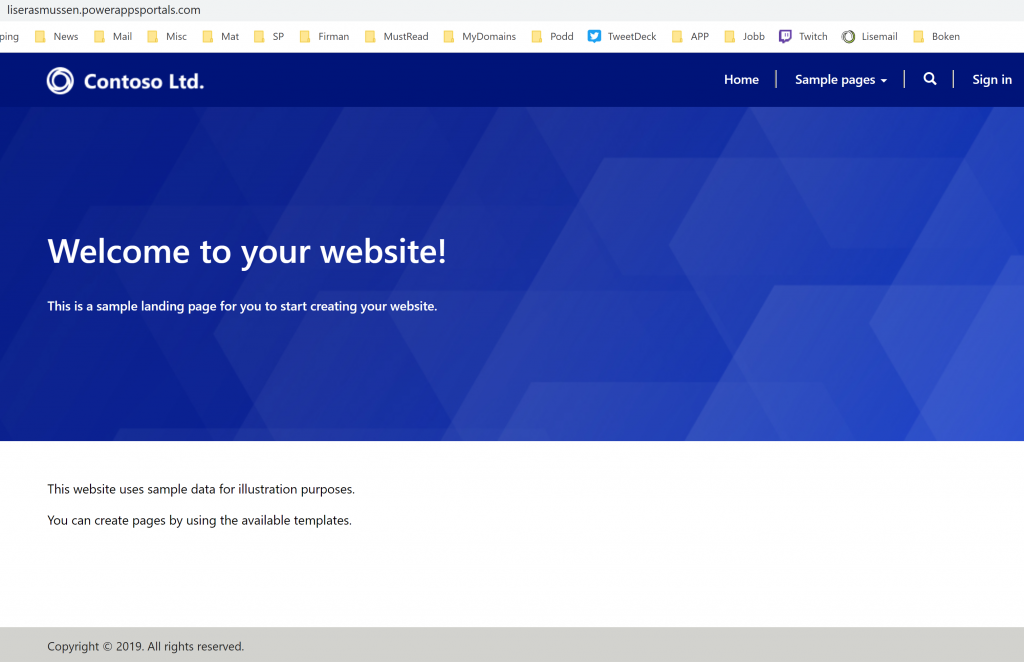The screenshot captures a website with the URL luceramucin.powerappsportals.com. The browser displays numerous bookmark tabs labeled as News, Mail, Music, Matt, SP, Firman, Must Read, My Domains, Pod, Twitter Deck, App, Jab, Twitch, LeaseMail, and Boken. The website's title, "Contoso Ltd," is prominently displayed on the left side of the header. On the right side, there are navigational elements including a Home tab, a drop-down menu titled "Sample Pages," a search icon, and a Sign In tab. Just below this header, the site welcomes users with the text, "Welcome to your website. This is a sample landing page for you to start creating your website." Further down, it adds, "This website uses sample data for illustration purposes. You can create pages by using the available templates."